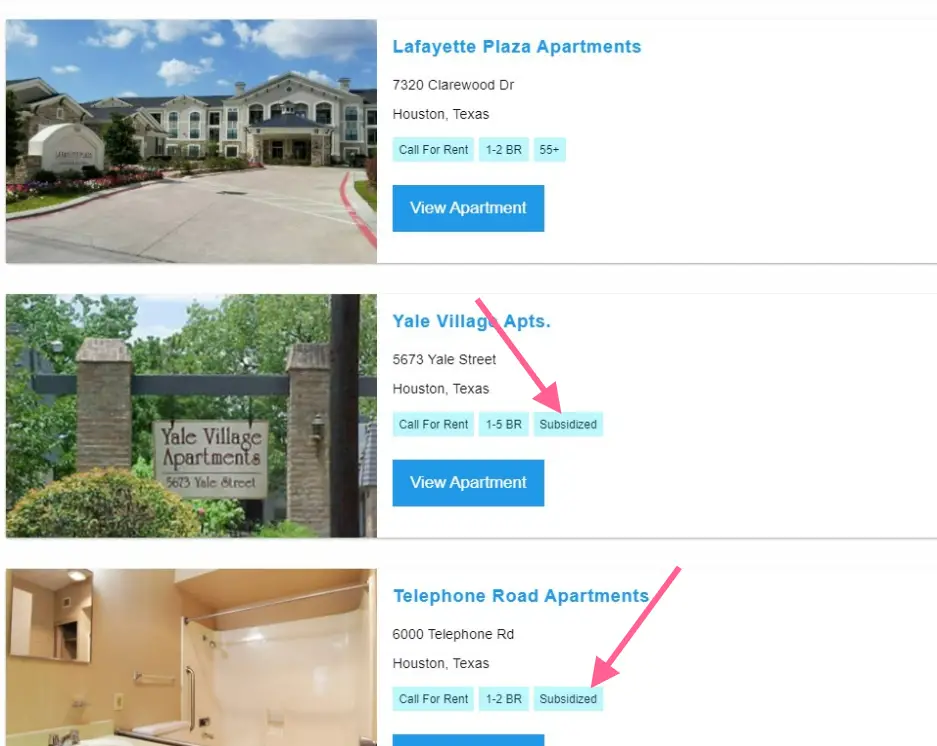The image showcases three apartment listings in a stacked format, likely from a real estate website or rental application. 

1. The first listing features Lafayette Plaza Apartments, located at 7320 Clarewood Drive, Houston, Texas. This listing includes a button labeled "Call for Rent," indicating that pricing details are available upon inquiry. The apartments offer between 1 to 2 bedrooms and are designated for residents aged 55 and older. A blue "View Apartments" button invites viewers to explore further. To the left of this listing is a photograph depicting the front of the Lafayette Plaza Apartments building.

2. The second listing is for Yale Village Apartments, situated at 5673 Yale Street, Houston, Texas. Similar to the first listing, it has a "Call for Rent" button for obtaining rental information. These units range from 1 to 5 bedrooms. A red arrow highlights the word "Subsidized," suggesting that rental subsidies may be available for eligible tenants.

3. The third listing advertises Telephone Road Apartments, located at 6000 Telephone Road, Houston, Texas. This listing also features a "Call for Rent" button, indicating that potential renters need to contact for pricing. The apartments offer between 1 to 2 bedrooms and include a "Subsidized" label, emphasized by a red arrow to underscore the availability of financial aid for qualifying residents.

Each listing provides a combination of key details and visual cues to assist prospective renters in making informed decisions.